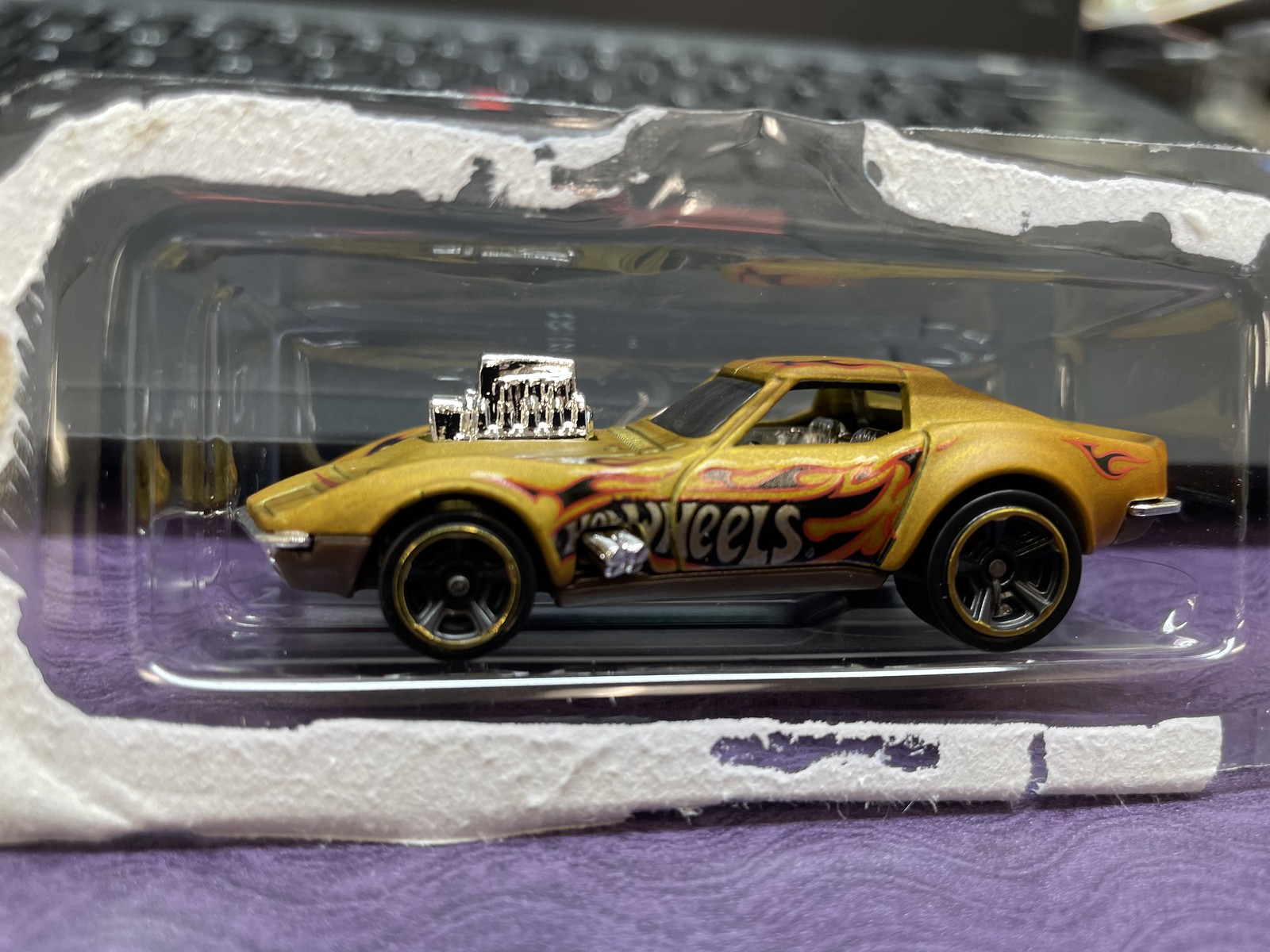The image depicts a vintage Hot Wheels toy car still in its original packaging, albeit opened and turned upside down. The car itself is a vivid gold color with striking red and black flames adorning the driver's side door and roof. A prominent sticker on the car proudly displays the iconic Hot Wheels logo. Adding to its classic, race-inspired design, the car features an oversized engine on top, reminiscent of old-school race cars. The clear plastic packaging shows signs of age, suggesting the toy hasn't been touched in a long time. This nostalgic piece is photographed on a purple surface, possibly a carpet or table, highlighting its display nature.